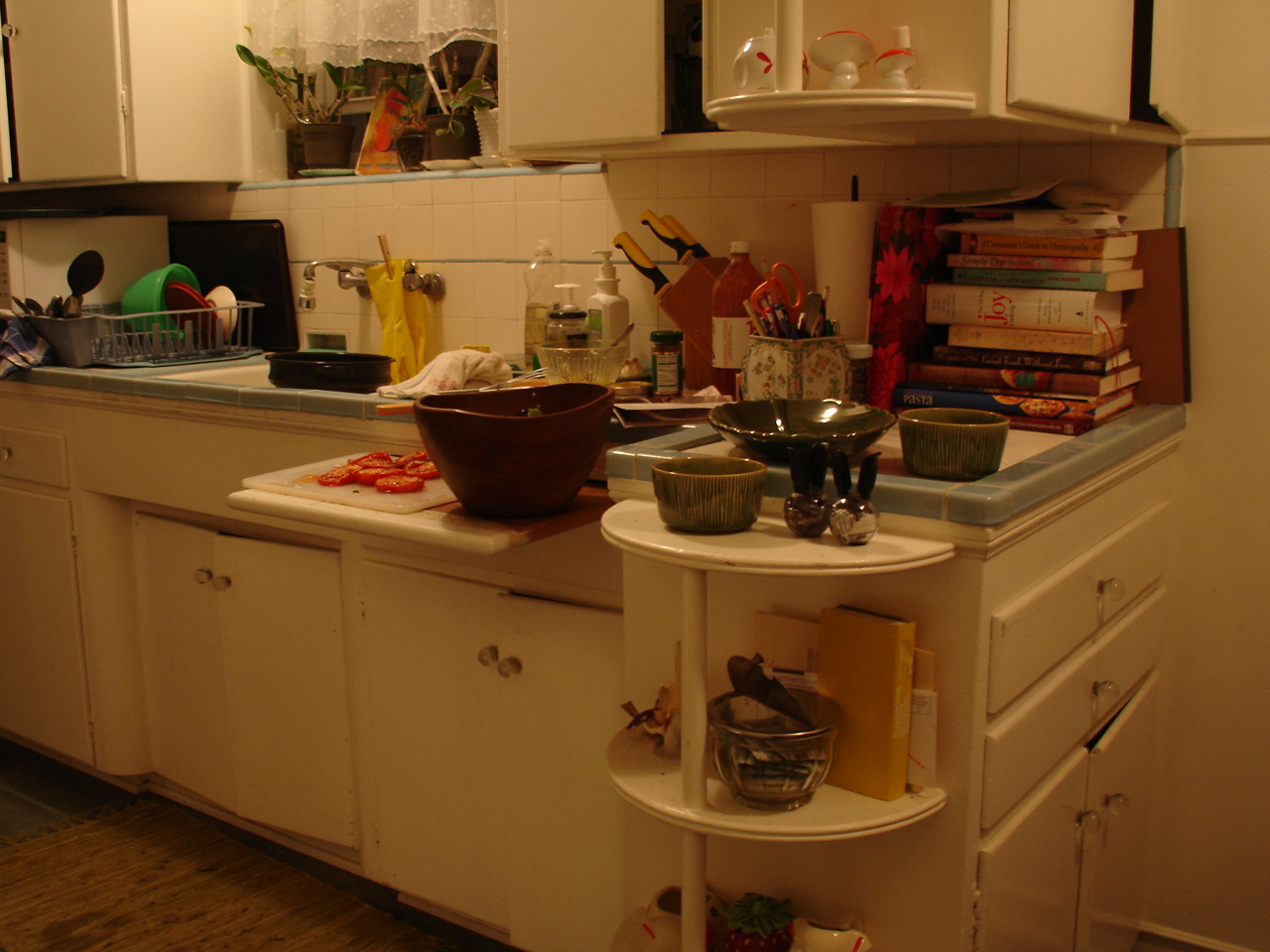In this vibrant kitchen scene, a meticulously organized stack of books stands at the far end of a countertop. Along the base of the counter are white cabinets with sleek door handles, which extend into drawers on the right-hand side. The countertop itself is tiled, providing a rustic yet clean surface. Amidst the books, one titled "Joy" in a white cover stands out. A metal bowl sits nearby, alongside a jar filled with ceramic utensils and scissors, a roll of toilet paper, and a wooden block with an array of knives. The backsplash features pristine white tiles, complemented by a small window with a white curtain that lets in natural light. Centered perfectly below the window, a metal faucet adorned with a hint of yellow rubber adds a touch of modernity. The drying rack is neatly arranged with bowls and utensils, while a white cutting board holds seven neatly sliced tomato pieces, positioned next to another bowl, ready for culinary use.